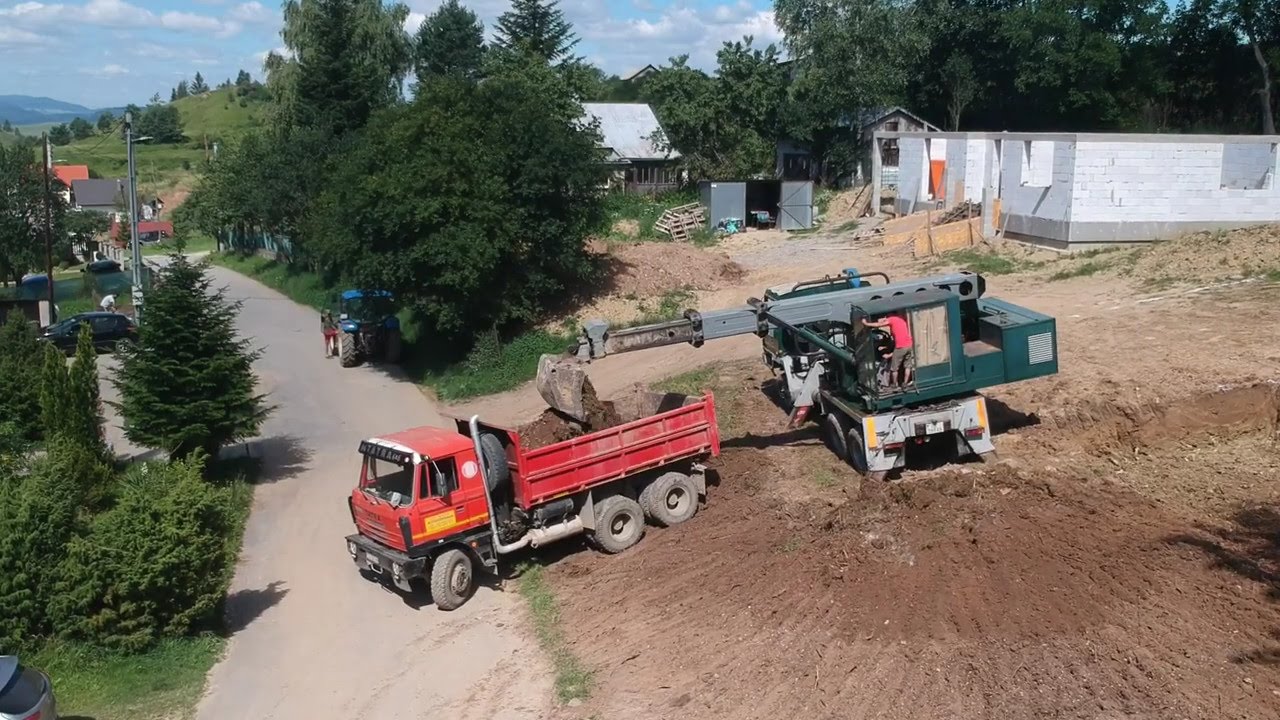In this daytime photograph, we observe a bustling construction site predominantly situated on the right two-thirds of the frame. The field is being cleared, revealing a vast expanse of brown dirt. Central to the field is a green tractor-like machine with a large scoop, actively loading dirt into a red flatbed truck positioned nearby. This red truck appears to be carrying both dirt and a large boulder. To the upper right, the cement foundation and the beginnings of a house are visible, depicting a hollowed-out structure in its early stages of construction. The background features numerous evergreen trees, alongside other trees with green leaves, painting a backdrop of natural beauty under a blue sky adorned with white clouds.

To the left side of the photograph, there's a long, light brown road that stretches from the bottom toward the top of the image. Flanked by grassy areas and additional trees, this road leads past several small houses nestled amongst the greenery. The setting suggests a small-town construction scene, with the road and residential structures contrasting against the industrial activity occurring in the foreground.